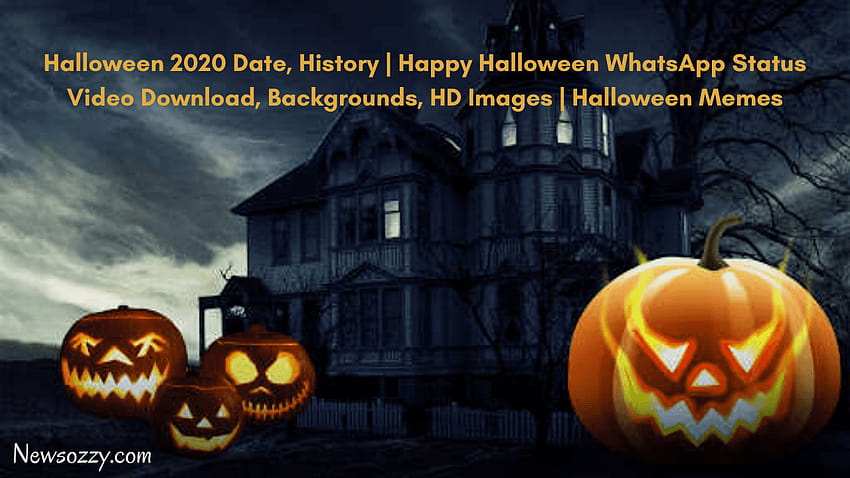This rectangular image, oriented horizontally, serves as an advertisement for Halloween. The top portion features the words "Halloween 2020: Date, History, Happy Halloween, WhatsApp Status, Video Download, Backgrounds, HD Images, Halloween Memes" in vivid orange text. The bottom left corner is marked with the URL "NewsAussie.com."

The background enhances the eerie atmosphere with a black and gray depiction of a haunted house, complete with a few dimly lit windows amidst predominantly darkened ones. A dead, leafless tree stands ominously to the right of the house, under an overcast sky thick with clouds, adding to the spectral ambiance.

In the foreground, the image is populated with ominous pumpkins. To the right, a jack-o'-lantern stands alone, its eyes and mouth emitting eerie smoke or flames. On the left side, three other jack-o'-lanterns with variably sinister expressions contribute to the spooky scene, each carved with slightly different menacing faces. This composition skillfully combines textual content with a haunting visual backdrop, capturing the quintessential Halloween spirit.